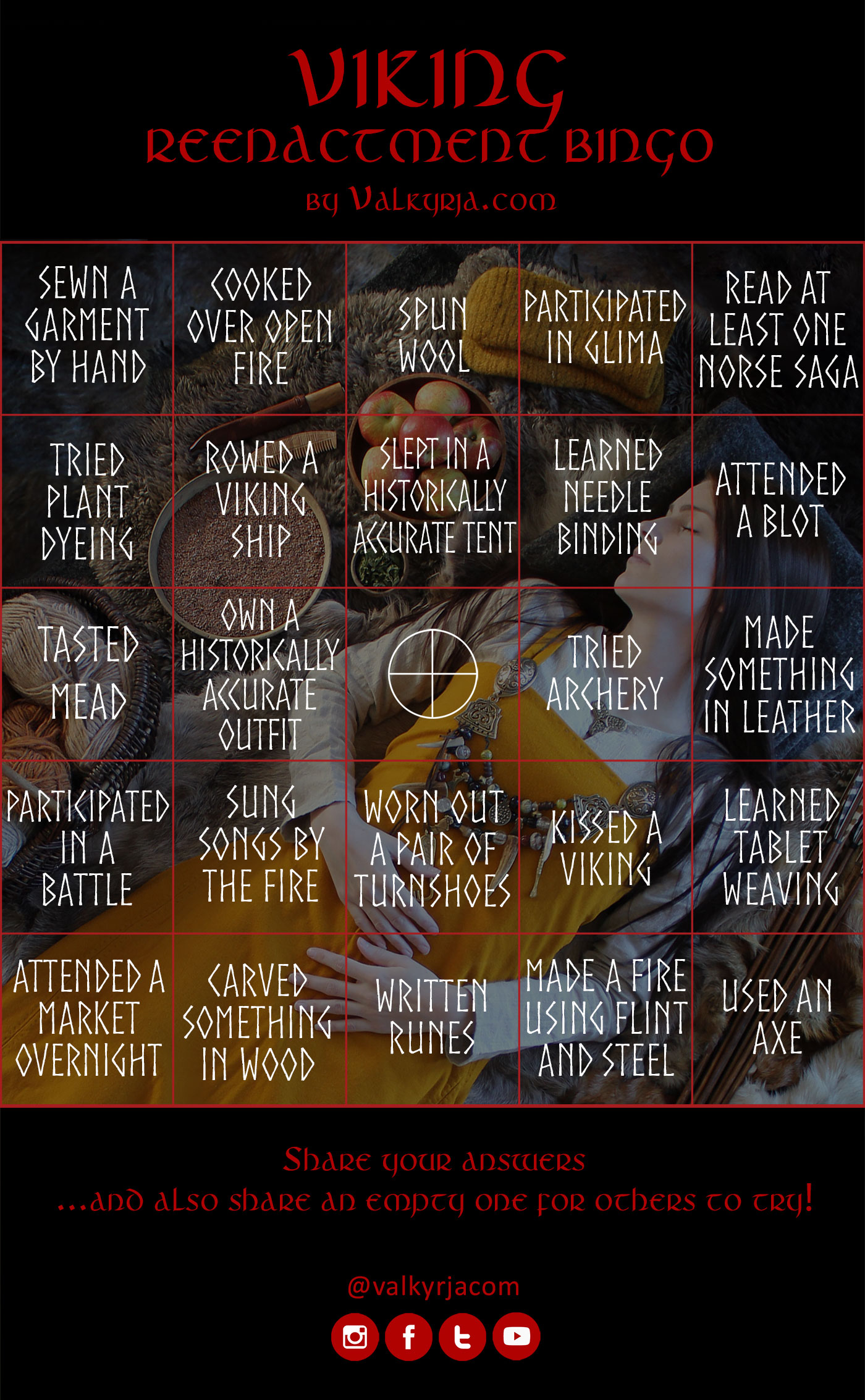This captivating vertical image serves as a bingo card for Viking reenactment enthusiasts. The image features a black background with bold red text at the top that reads "Viking Reenactment Bingo" and additional red text at the bottom instructing viewers to "share your answers and also share an empty one for others to try." The bottom also includes social media icons in red circles and the website "valhalla.com."

The focal point of the image is a realistic photograph of a Viking woman lying on her back, dressed in a red dress with a white shirt underneath. Her dark hair falls around her head, which is slightly turned to the left, and her hands rest on her stomach. Surrounding her are traditional Viking foods like bread, apples, and rice.

Overlaying this scene is a 5x5 bingo board with 25 white-font squares. Examples of activities listed in these squares are "used an axe," "tried archery," "written runes," "tasted mead," "spun wool," "tried plant dyeing," "attended a blot," "attended a market overnight," "carved something in wood," "participated in glima," "read at least one Norse saga," "made something in leather," "sewn a garment by hand," "rode a Viking ship," and "sung songs by the fire." The center bingo piece features a distinct white circle with a vertical and horizontal line intersecting to form a plus sign. This richly detailed image not only captivates the eye but also invites participants to engage in Viking culture through an interactive and educational activity.